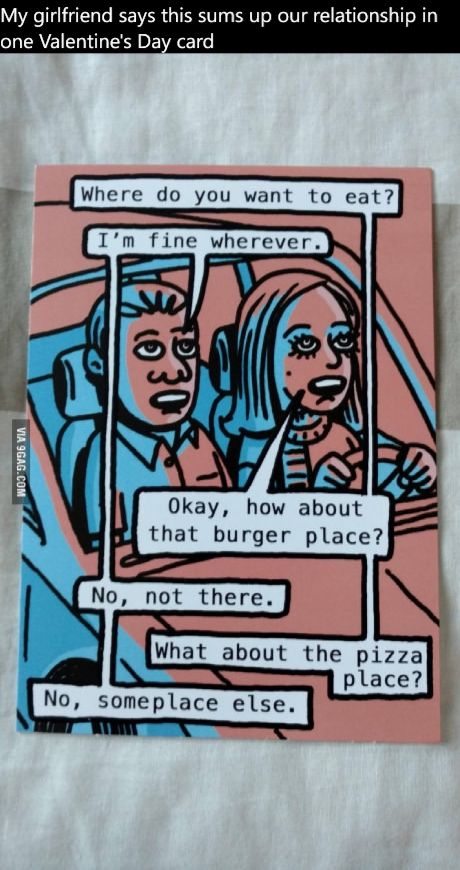The image is a tall, rectangular Valentine's Day card placed against a white fabric surface. Across the top of the image is a black bar with white text that reads, "My girlfriend says this sums up our relationship in one Valentine's Day card." The card itself features a cartoon in shades of pink and blue with black outlines, depicting a woman and a man in a car. The woman, who is driving, is on the right, while the man sits in the passenger seat. Their conversation is shown in speech bubbles: 

- Woman: "Where do you want to eat?"
- Man: "I'm fine wherever."
- Woman: "Okay, how about that burger place?"
- Man: "No, not there."
- Woman: "What about the pizza place?"
- Man: "No, someplace else."

The site watermark "va9gag.com" is visible on the card. The comic humorously illustrates a common relationship scenario where indecisiveness meets contradictory choices.